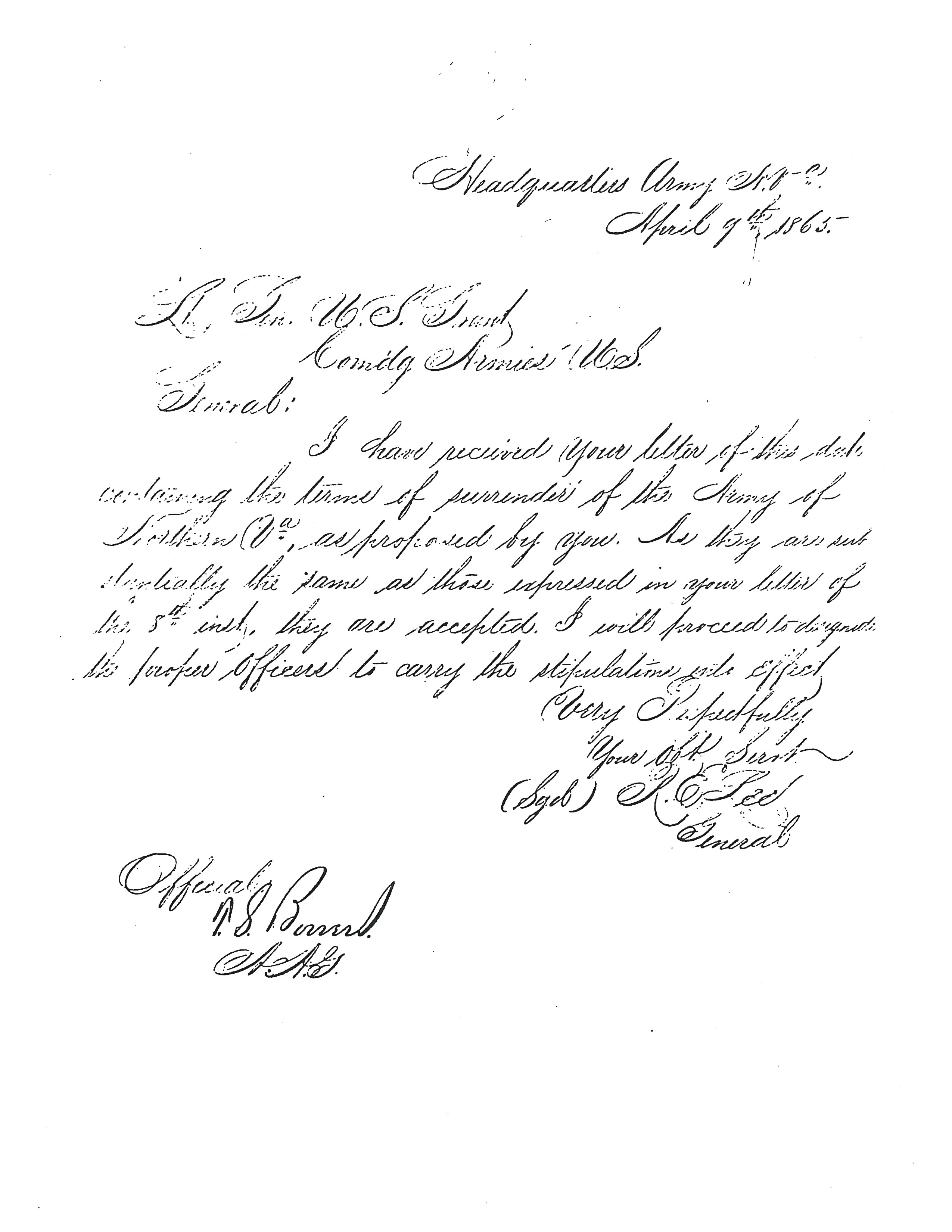This image features a letter set against a plain white background. The text, in cursive handwriting, is notably challenging to read due to its grainy, pixelated quality, suggesting it is a copied version. The handwriting is very loopy and ornate, making it even more difficult to decipher any specific words or phrases. At the top, there appears to be a date and possibly a name; hints of "April 9th, 1865" can be made out. Throughout the letter, fragmented words like "headquarters," "surrender," "U.S. Grant," and phrases such as "I have received your letter" are somewhat recognizable but incomplete. The content is largely illegible, marked by numerous interruptions and gaps in the text. A signature, again too blurred to read clearly, is located at the bottom left of the letter, adding to its historical and military context suggested by the mention of "Sergeant." Overall, the letter's contents remain elusive due to the poor quality of the reproduction.